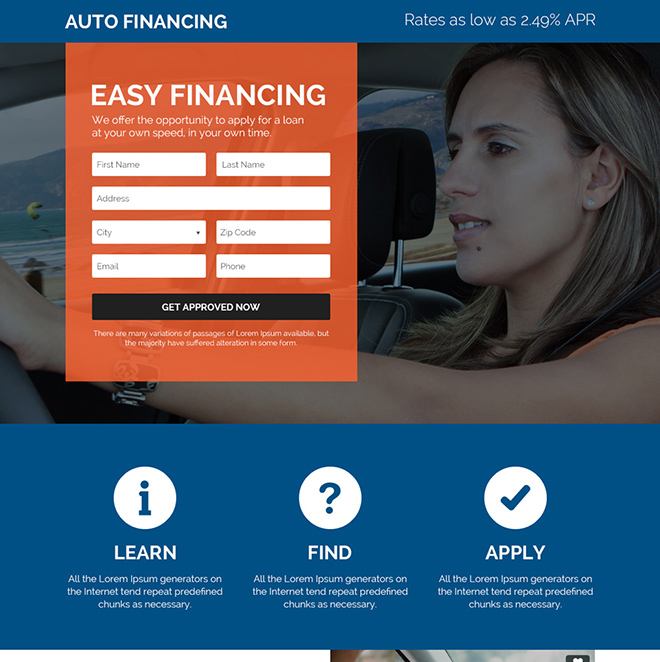This image is a website template from a popular website builder platform, characterized by placeholder text, "lorem ipsum," used throughout. The template appears to be designed for an auto financing service. 

At the top, there is a blue bar with white block text on the top left that reads "Auto Financing," and thinner white text on the top right indicating "Rates as low as 2.49% APR." 

Below this bar, an image of a Caucasian woman with brown hair is shown, seated in the driver’s seat of a car, facing left, and appearing deeply focused. The image is intentionally faded, serving as a background rather than the focal point.

The primary focus of the template is an orange box on the left side, featuring large white text that reads "Easy Financing." Beneath it, smaller white text states, "We offer the opportunity to apply for a loan at your own speed, in your own time." This section contains seven user input fields labeled: Name, First Name, Last Name, Address, City, Zip Code, Email, and Phone Number. Centered below these fields is a black button with white text that says "Get Approved Now." Further down, in very small white text, is the placeholder filler text indicating modifications from the original lorem ipsum text.

The lower third of the image contains another blue section matching the top bar's color. This section features three equidistant icons. The first icon, a circle with a lowercase "i" in the center, is labeled "Learn," accompanied by more lorem ipsum text. The center icon, a blue circle with a white question mark, is labeled "Find" in large white text. The rightmost icon, another circle containing a checkmark, is labeled "Apply."